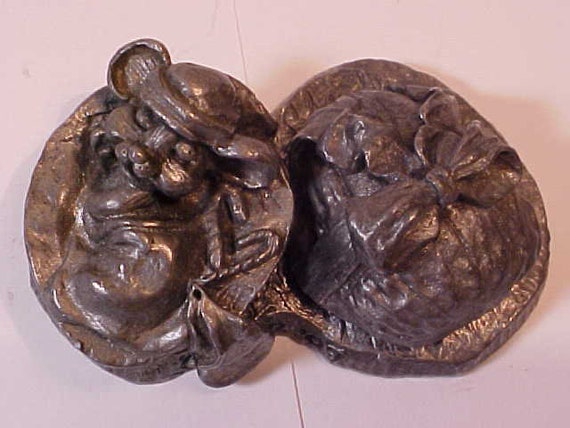This detailed image showcases an intricately crafted wooden carving, split into two distinct oval sections joined seamlessly at the center. The piece is flat and doesn't fold, highlighting the artisan's skill in relief carving. The left side of the artwork features two prominent faces—the uppermost resembling a cat adorned with a playful hat, while the lower one appears to be a mysterious mask. The right side presents a different motif, possibly depicting a flowing plant or a delicate ribbon tied into a bow. The craftsmanship is evident in the deep carving, showcasing the meticulous chisel marks where the wood has been expertly gouged and removed. The detail and texture bring the carved figures to vibrant life, making this piece a compelling study of traditional wood carving techniques.